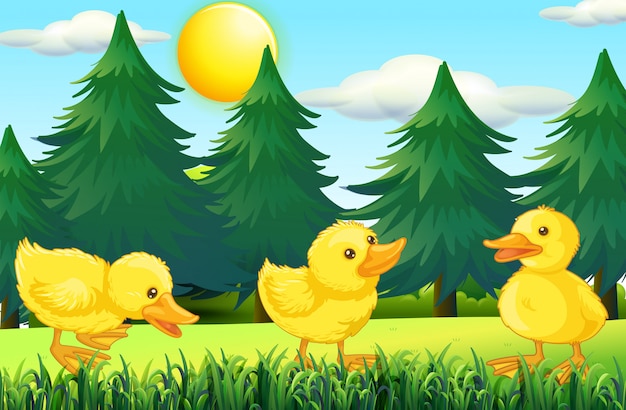The image is a vibrant, cutesy cartoon scene reminiscent of a children's book, featuring three yellow ducklings with dark yellow, almost orangish beaks, legs, and cute little black eyes. The ducklings are positioned on a flat, green grass plane with some short grass in front of them, and a layer of taller grass behind them. The duckling on the far left is bending down and looking to the right with its mouth open, the center duckling also looks to the right with a closed mouth, and the rightmost duckling faces left with an open mouth. The background showcases a picturesque field with a bunch of cartoon pine or evergreen trees with brown trunks and some green bushes. Above the trees, a turquoise blue sky is dotted with fluffy white clouds that have shaded undersides for depth. A large, bright yellow sun shines in the top center-left of the scene, lighting up the entire joyful tableau. The art style is characterized by solid colors without outlines, shaded for texture and depth, creating a warm and delightful atmosphere.